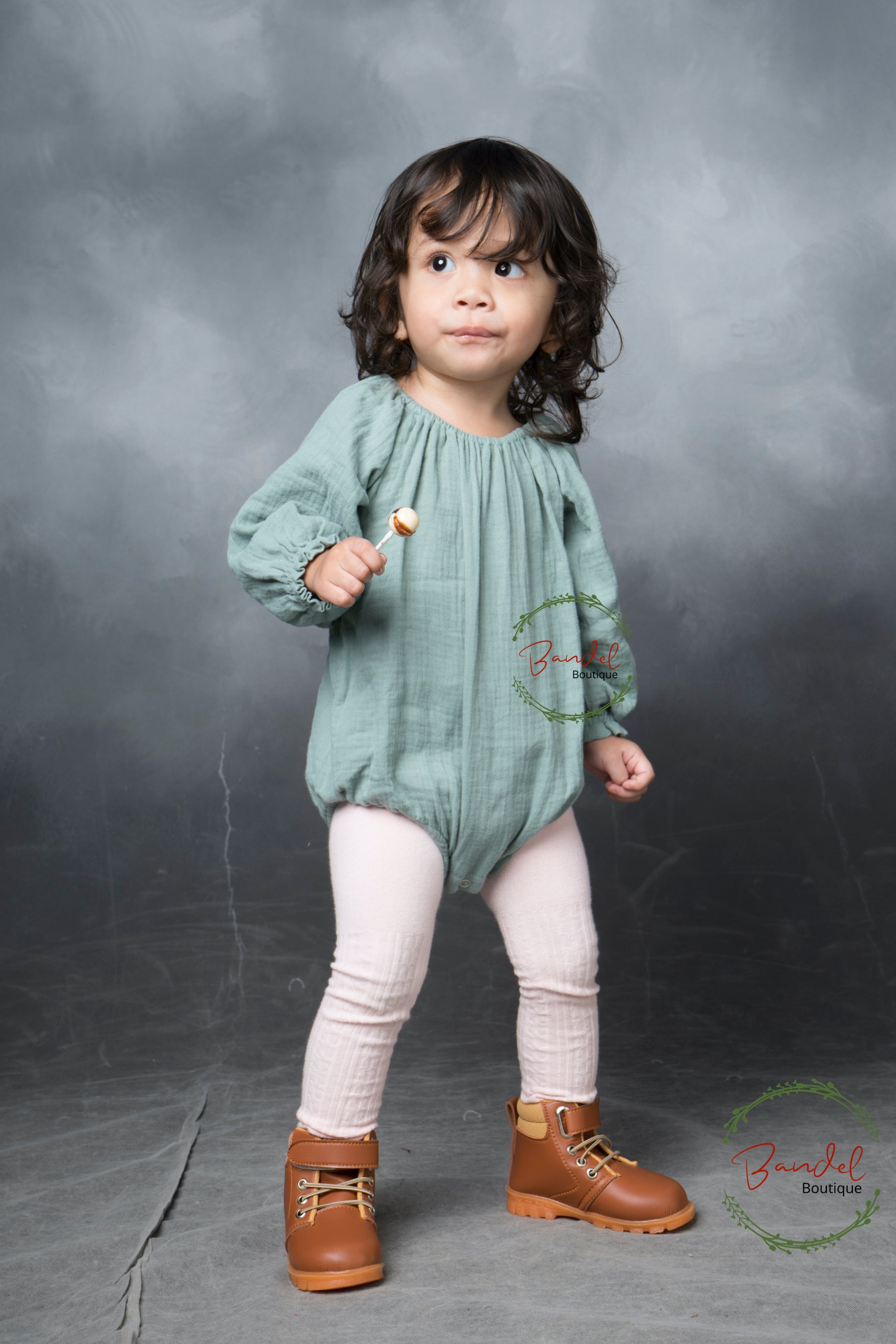This professionally shot photograph captures a young girl standing against a smoky, gray, and cloudy backdrop, evocative of a glamor shot. The toddler, with her long, curled black hair draped over her shoulder, possesses big brown eyes and is smiling while holding a distinctive lollipop—a white ball with a brown stripe—in her hand. She is dressed in a pale sage green, long-sleeve onesie paired with white tights, and her feet are adorned with caramel-colored leather boots featuring velcro straps. The bottom right of the image is branded with the Bandle Boutique logo, characterized by green olive leaves forming a wreath and dark red-orange lettering for "Bandle" with "Boutique" in black beneath it.